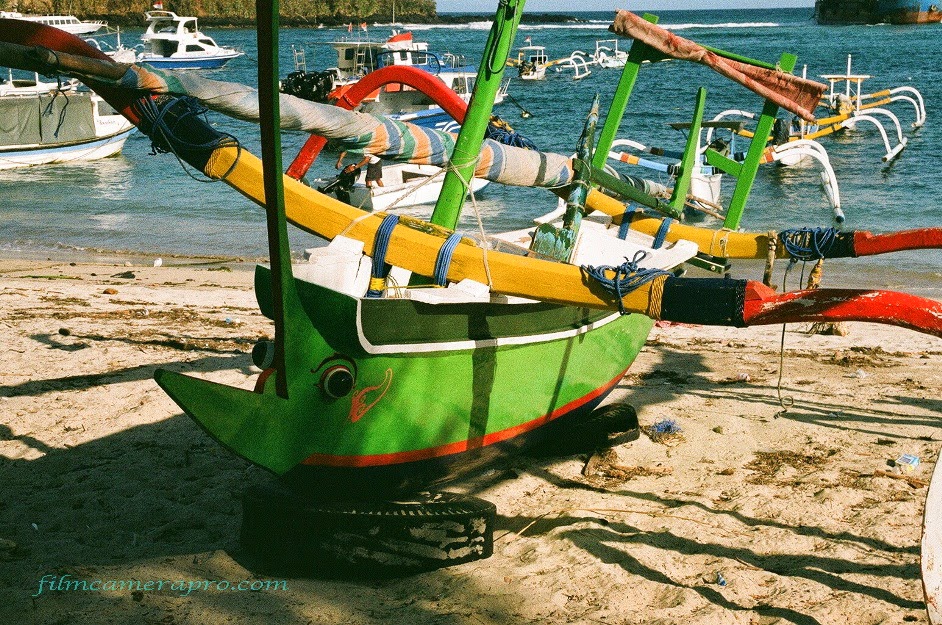This photograph captures a busy beach scene with various watercraft, some of which have been creatively modified. In the foreground, there is a small green boat with a unique design. It has a pointed front resembling a nose, and two black circles that imitate eyes, giving it an animalistic appearance, almost like a reptile. The boat features a red stripe along the bottom, a dark blue stripe beneath that, and has yellow, black, and red components attached across the top that seem like floating arms. The boat rests on black tires embedded in the sand.

In the background, the ocean stretches out with several other water vehicles that have white legs extended from their sides, suggesting pontoons for balance. Some of these boats also display yellow coloring. To the left, there is a larger motorized boat with blue and white coloring. The overall setting indicates it is daytime, as evidenced by the shadows on the sand.

The scene includes an image's bottom left corner marked with "FilmCameraPro.com" in blue font. The photo, with its mix of creative and standard boats, evokes a sense of whimsical clutter against the natural backdrop of the beach and ocean.